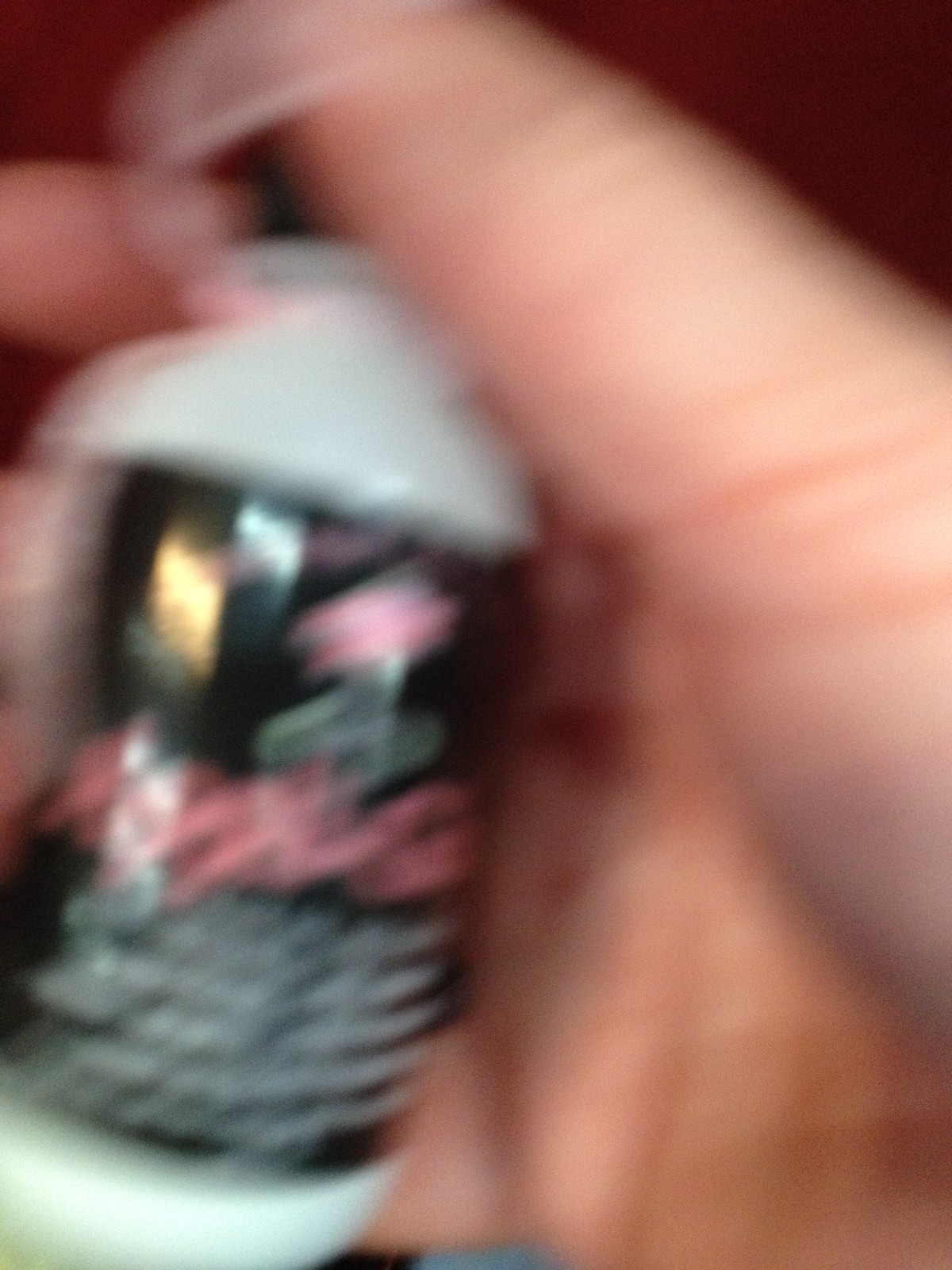In this extremely blurry, close-up image, there's a right hand, appearing to be male, holding a small, cylindrical bottle. The bottle itself is predominantly milky white with a black cap and a black label. Centered on the label is an icon featuring gold hues in the top-left corner. Below this, the label displays pink and white script, with a prominent light pink title followed by several lines of smaller white text. The hand is positioned directly facing the viewer, with the thumb on the cap and the index finger beneath it, while the bottle rests against the palm and is supported by the middle, ring, and pinky fingers. The hand reveals some wrinkles, noticeable mainly in the lower center right area, adding depth through visible shadow lines. Despite the overall blurriness, it's evident that the hand is holding a bottle, potentially a vitamin or medicine container.